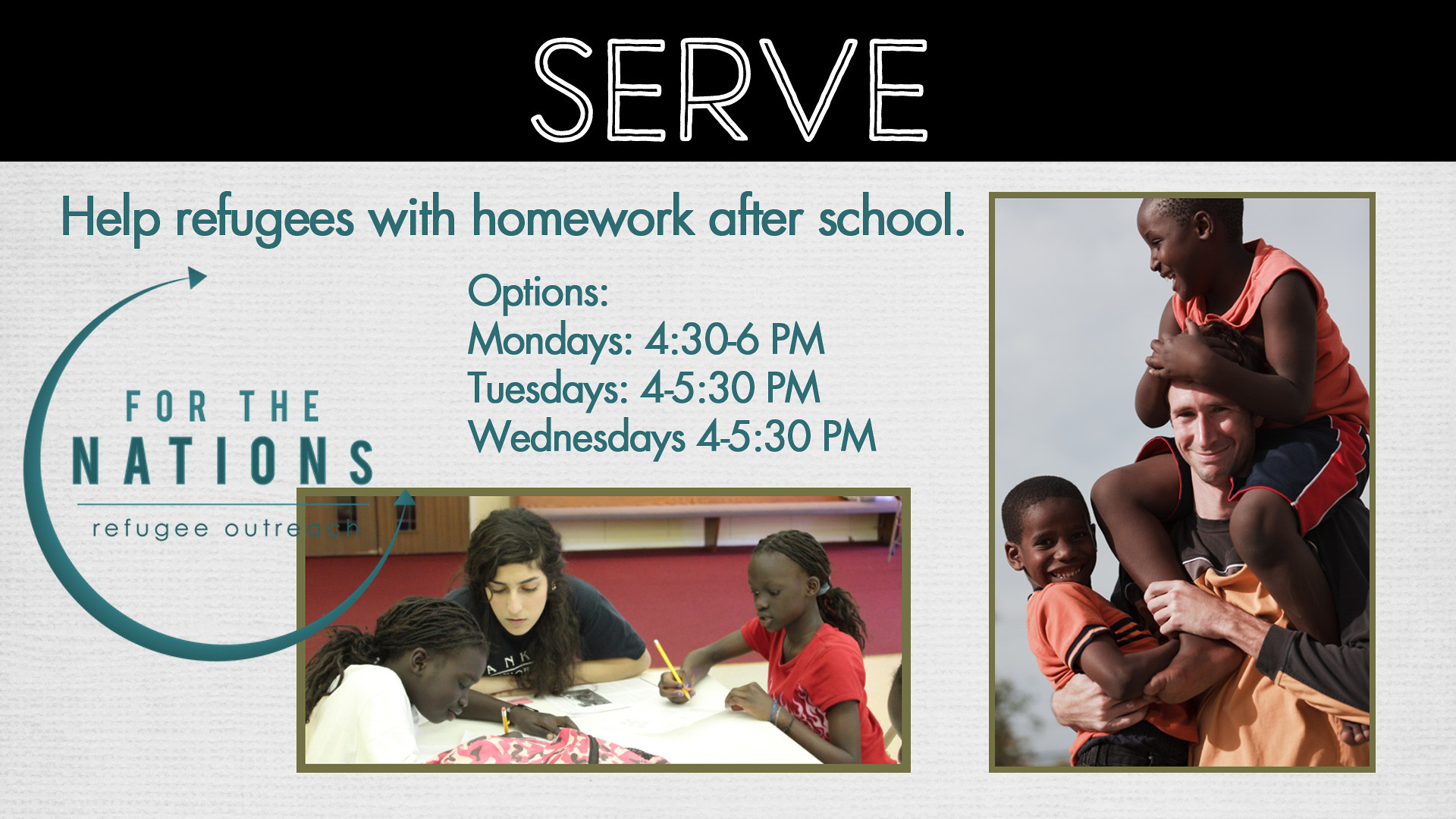This image features a rectangular, computer graphic wider than it is tall. At the top, a black horizontal strip spans the width of the image, containing the word "SERV" in bold white letters. Below this header, the background changes to a light gray. Centered in blue text, a message reads: "Help refugees with homework after school. Options: Mondays 4:30-6:00 p.m., Tuesdays 4:00-5:30 p.m., Wednesdays 4:00-5:30 p.m."

On the left side of the image, there's a circular logo with the text, "For the Nations, Refugees, Outreach." Beneath the text is a detailed photograph showing a white woman assisting two African children with their homework around a table in a room setting. On the right side of the image, there is another photograph, this time depicting a Caucasian man smiling while holding two African boys—one in his arms and one on his shoulders. Both boys are smiling and wearing red shirts. Overall, the image emphasizes the supportive, educational, and community-oriented environment provided by the SERV program.